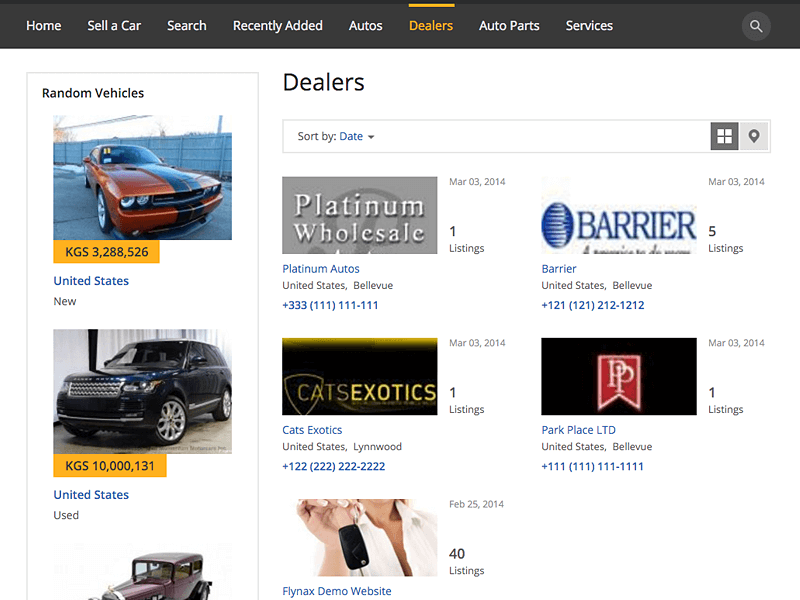This is a detailed description of a screenshot from an online car selling platform. The topmost section of the screenshot features a black navigation bar with the following white text options: "Home," "Sell a Car," "Search," "Recently Added," "Autos" (highlighted in orange), "Auto Parts," "Services," and a search button.

Beneath this, the interface has a white background displaying several car images on the left. Among these images are a red and blue vintage car bearing the logo "KGS3288526," labeled as "United States new," and a black car marked "KG100131," labeled as "United States used." Notably, the top car in the image gallery appears to be a dark maroon vintage car from the 1930s or 1940s, with no further details visible.

To the right of the car images, there is a section dedicated to dealer information. It includes a sorting option titled "Sort by Date" with a dropdown menu. The dealers listed include:

1. **Platinum Wholesale**: One listing, a black and white website, possibly associated with the vintage car.
2. **Platinum Auto**: Located in Bellevue, United States, accompanied by a phone number.
3. **Car Exotics**: One listing, based in Lyingwood, contactable via phone.
4. **Ryan, Fly Depot Website**: Displays an image of a woman's head and neck holding a car key, featuring 40 listings.
5. **Barrier**: Located in Bellevue, United States, with five listings.
6. **Park Place Ltd**: Also based in Bellevue, United States, with one listing. The logo is a black rectangle with a small red flag, containing the initials "P.P."

This detailed description effectively captures the contents and layout of the online car selling platform's screenshot, making it accessible even to those unfamiliar with cars.